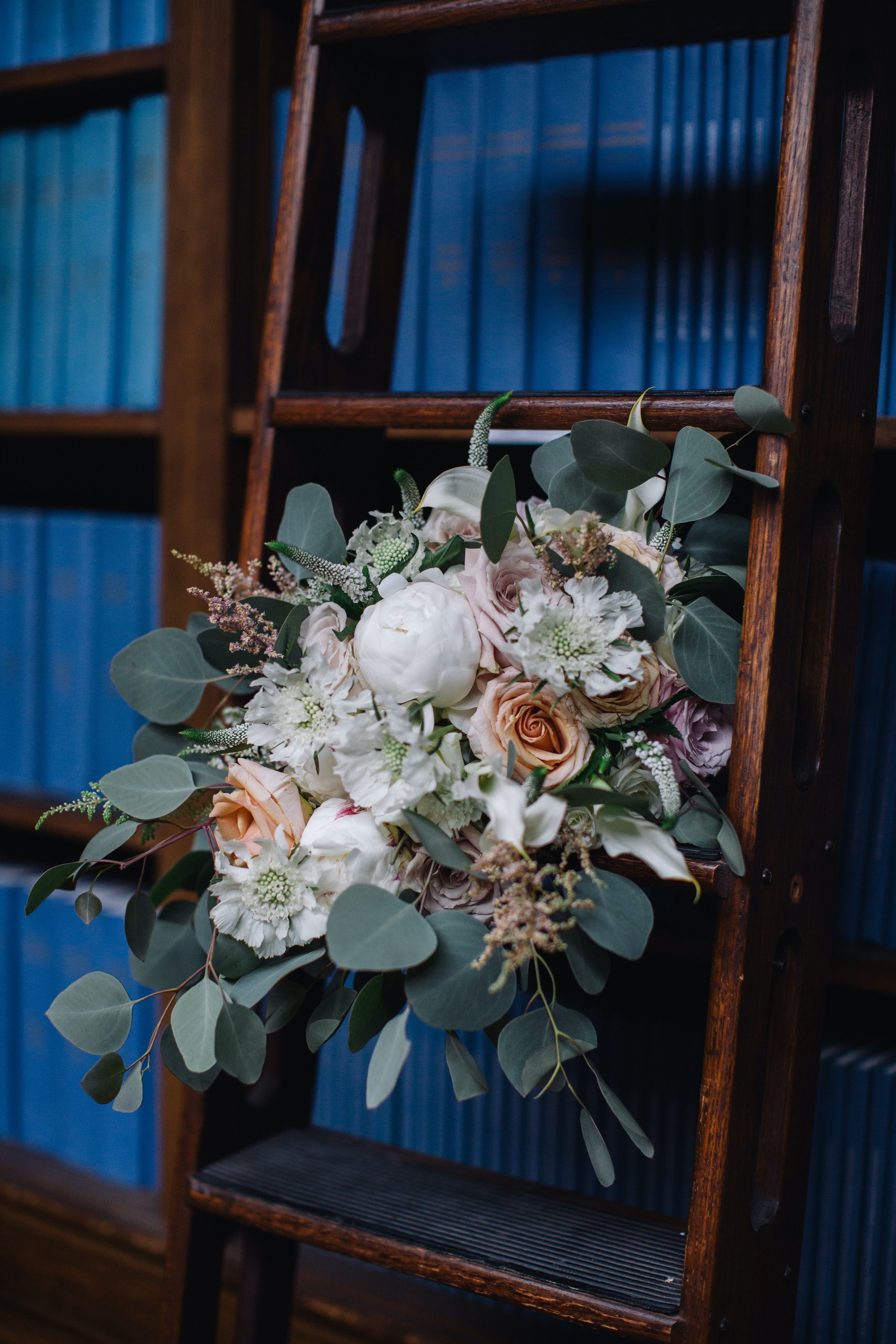The photograph captures a rich, dark wood-paneled room filled with rows of bookshelves. These bookshelves are meticulously packed with blue books, each adorned with gold lettering too small to decipher. All the books appear to be part of the same collection, with varying widths adding texture to the uniformity of their height. In front of one of these shelves stands a matching dark wood ladder, equipped with wheels to slide along the shelves. Perched on the second rung is a detailed bouquet of flowers. This bouquet features vivid orange roses, delicate white flowers, green leaves, and clusters of small, cocoon-like white blossoms interspersed with light purple blooms. The flowers are arranged in a way that they cascade naturally against the dark wood. Gentle shadows cast by the ladder and flowers create a play of light and dark on the richly hued shelves, adding depth and drama to the scene.